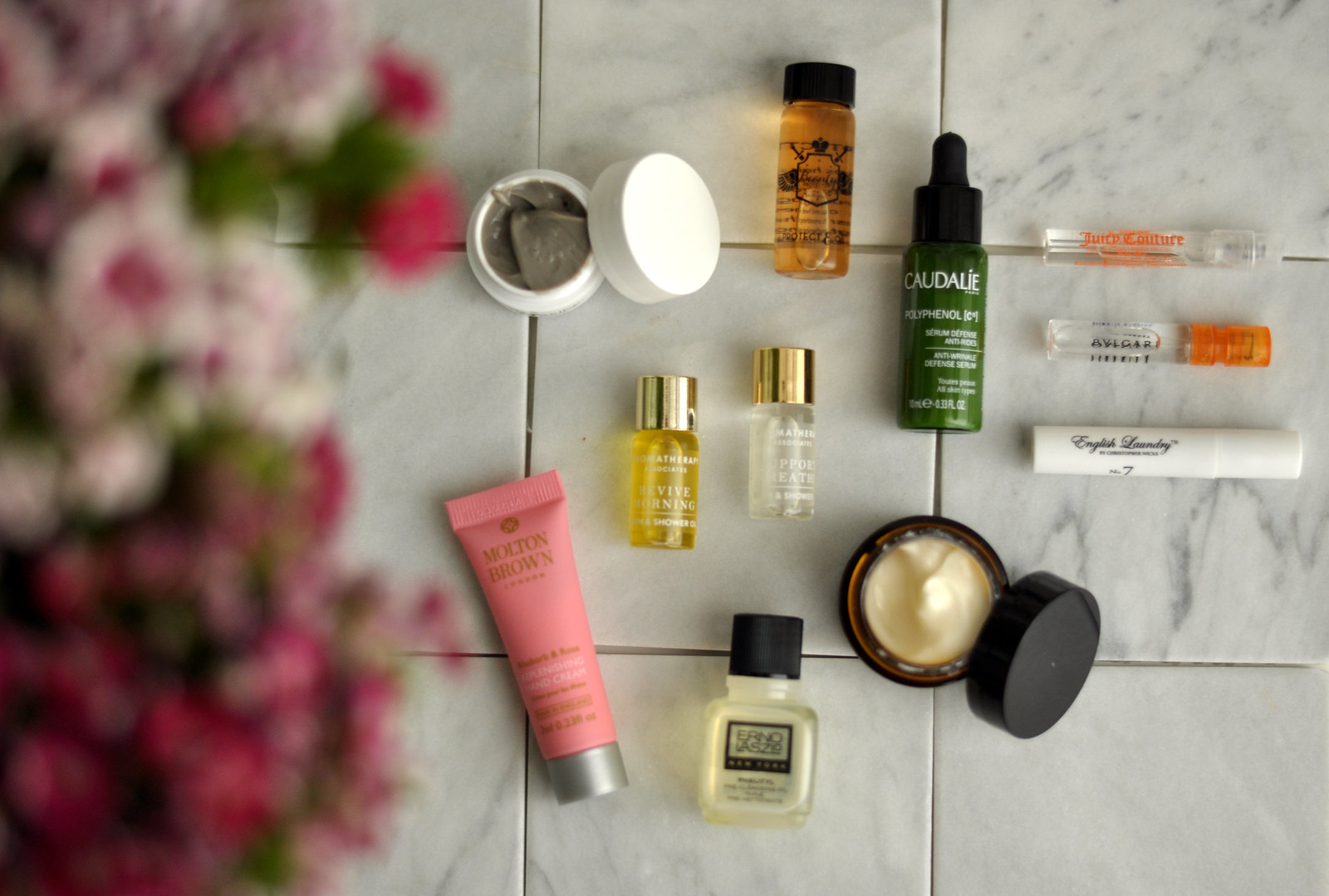The image showcases an array of makeup items meticulously arranged on a tiled surface. Dominating the scene is an open, circular black compact filled with a creamy white substance, suggesting it is a face cream or similar cosmetic product. Surrounding this central product are various bottles from different brands. Notably, there is a white case containing a gray-like substance, contrasting with the white cream in the compact.

Additionally, the image features approximately five clear vials. Among them, two are particularly small, two are slender, and one is of regular size, filled with a brown liquid. Next to this vial is a green, dropper-like bottle from Caudalie, emphasizing the variety of skincare items present. Adjacent to them is a bottle labeled "Molten Brown," which appears to be a squeeze bottle, likely containing lotion.

In the background, a softly blurred image of flowers adds a touch of elegance to the composition, all set against the clean, neutral backdrop of the tiled surface. This detailed arrangement highlights the diversity and functionality of the beauty products displayed.